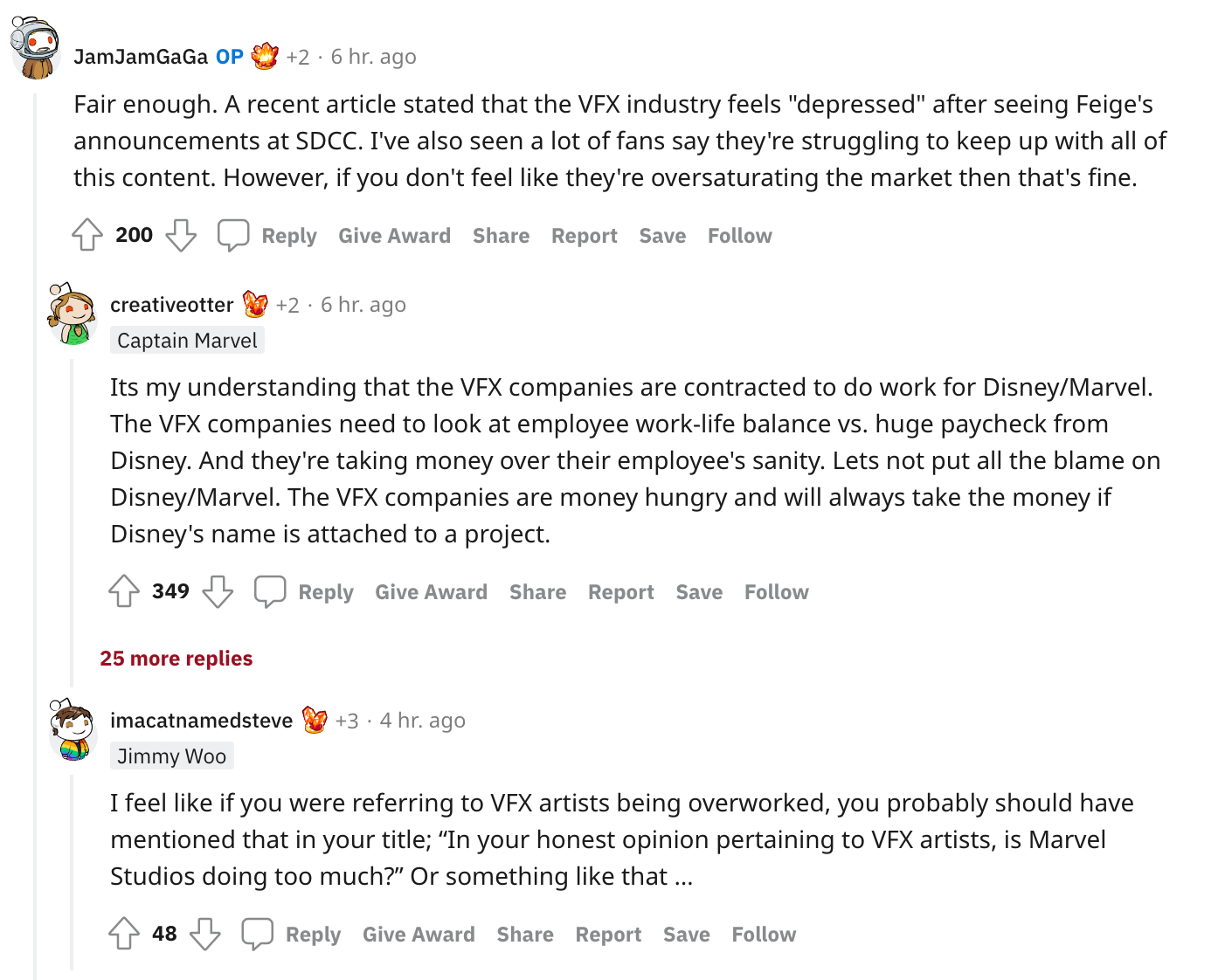The screenshot showcases a discussion thread on Reddit, focusing on the pressures faced by the VFX industry, particularly in relation to Marvel's projects. The background is white, and the text is black. The conversation starts with a comment from user JamJamGarGar, who notes that a recent article mentioned the VFX industry's sense of despair following Fage's announcements at SDCC, and highlights the struggle fans face in keeping up with the abundance of content. This comment has garnered 200 upvotes.

User CreativeOtter responds with a detailed critique, indicating that the VFX companies, contracted by Disney/Marvel, prioritize hefty paychecks over employee well-being, thus contributing to the industry's issues. CreativeOtter argues that while Disney/Marvel is partly to blame, VFX companies also play a significant role by choosing profit over their employees' sanity. This response has received 349 upvotes.

A further contribution comes from user I'mACatNameSteve, who suggests that if the discussion is about the overworking of VFX artists, it should be clearly mentioned in the title. They pose a question about whether Marvel Studios is overburdening VFX artists. This comment has received 48 upvotes.

The thread reflects an in-depth discourse on the work-life balance of VFX artists, the industry's financial motivations, and the responsibilities of major studios like Marvel.